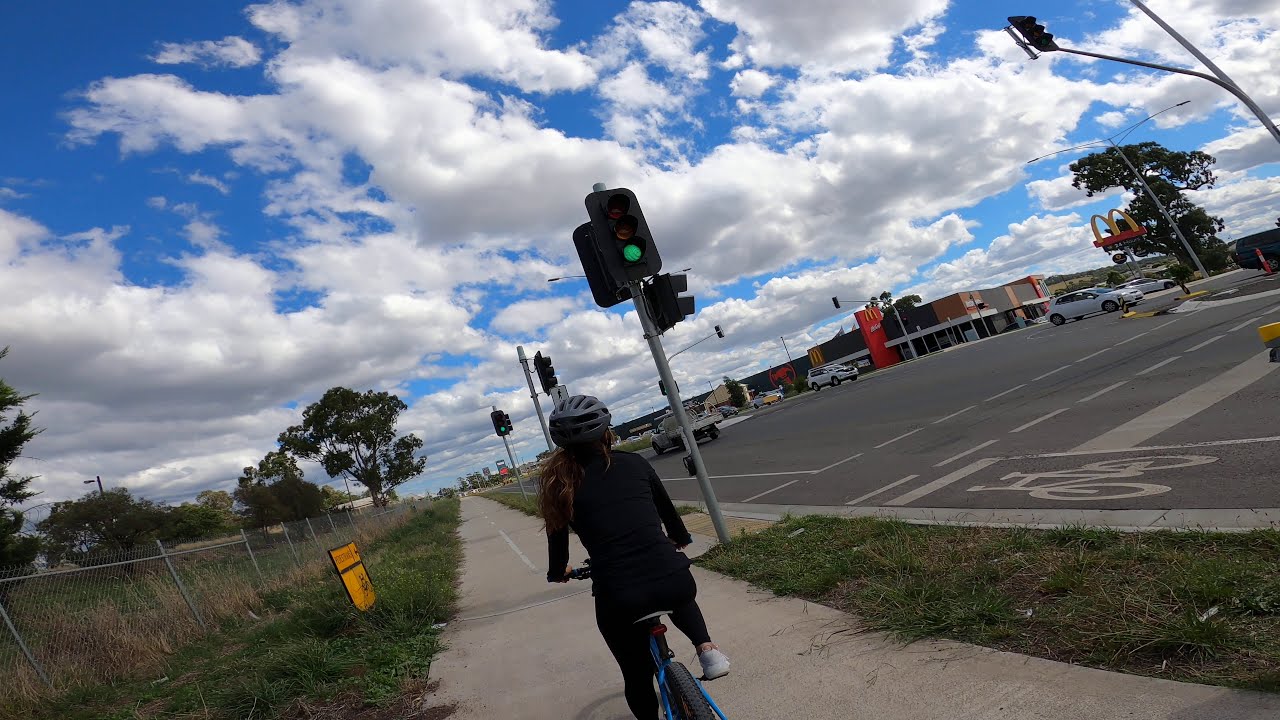In this outdoor cityscape scene, a woman riding a blue bicycle is prominently featured on a sidewalk that travels diagonally from the lower right to the middle left of the image. She is dressed in black leggings, a black shirt, and a black helmet. The sidewalk, clearly marked with white lines, is flanked by green grass and trees on the left. A silver metal mesh fence runs alongside the bike path on this side as well. 

In the foreground, a traffic light with a green signal presides over a crosswalk that she is approaching. The intersection ahead bustles with cars, including a few white cars and a truck, moving in both directions. On the middle right side of the image, a McDonald's restaurant adorned with its iconic golden arches is visible. The restaurant is situated near another traffic light located in the upper right-hand corner.

Above, the sky boasts a vibrant blue hue, interspersed with large, puffy white clouds. Trees dot the landscape in both the upper right and left corners, adding to the suburban ambiance of this busy area.